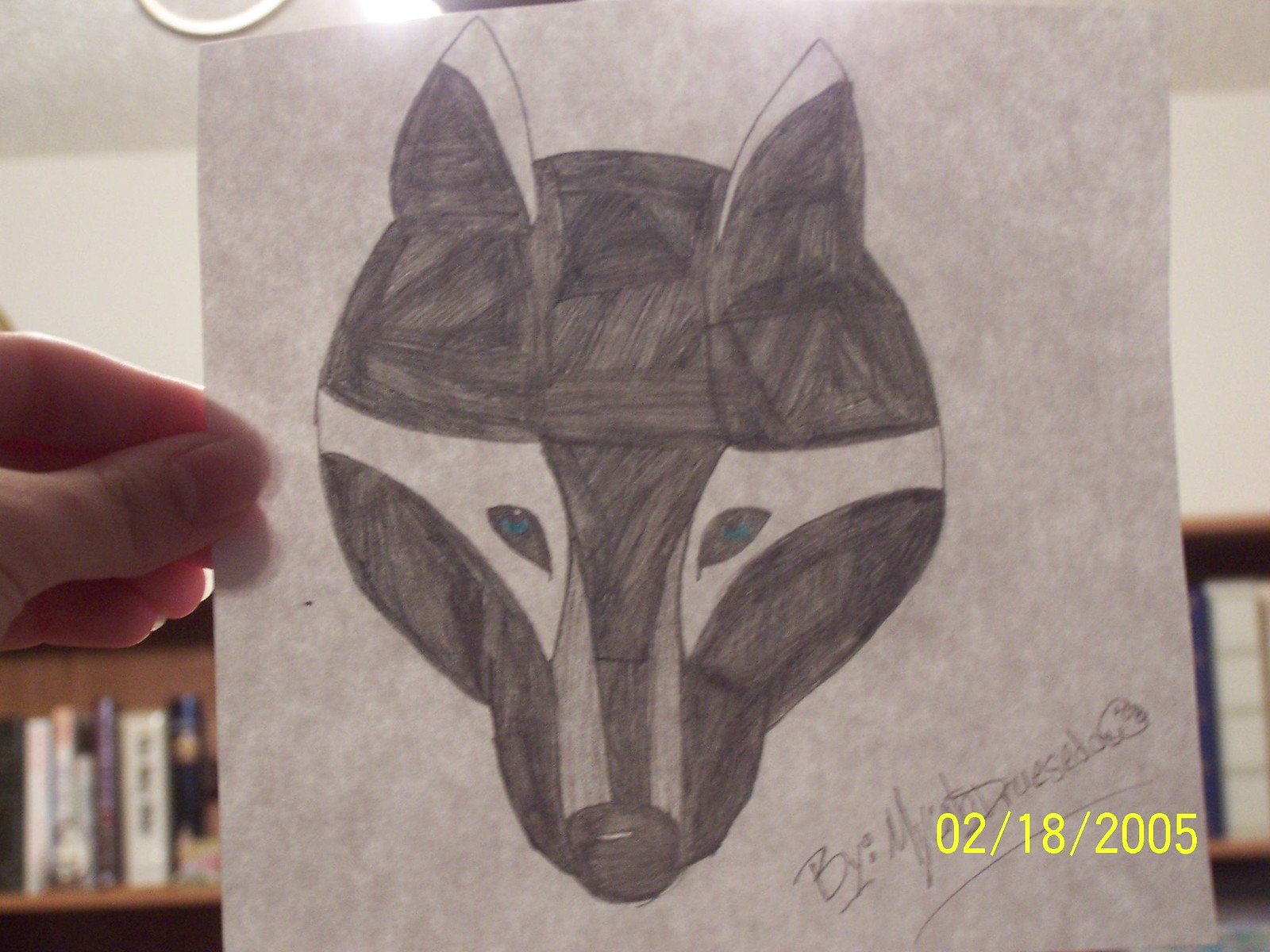The image captures a room with a light gray ceiling featuring a ceiling light fixture. The walls of the room are also light gray, creating a harmonious color palette. A wooden bookcase filled with numerous books is visible against one of the walls. In the foreground, a person's hand is holding a white piece of paper. The paper displays a detailed drawing of a fox. The fox's face is predominantly black, with lighter gray shading around its eyes and the sides of its nose. The tips of its ears are accented with white or light gray. The fox has striking deep blue eyes that draw attention. The drawing is signed and dated "02-18-2005."